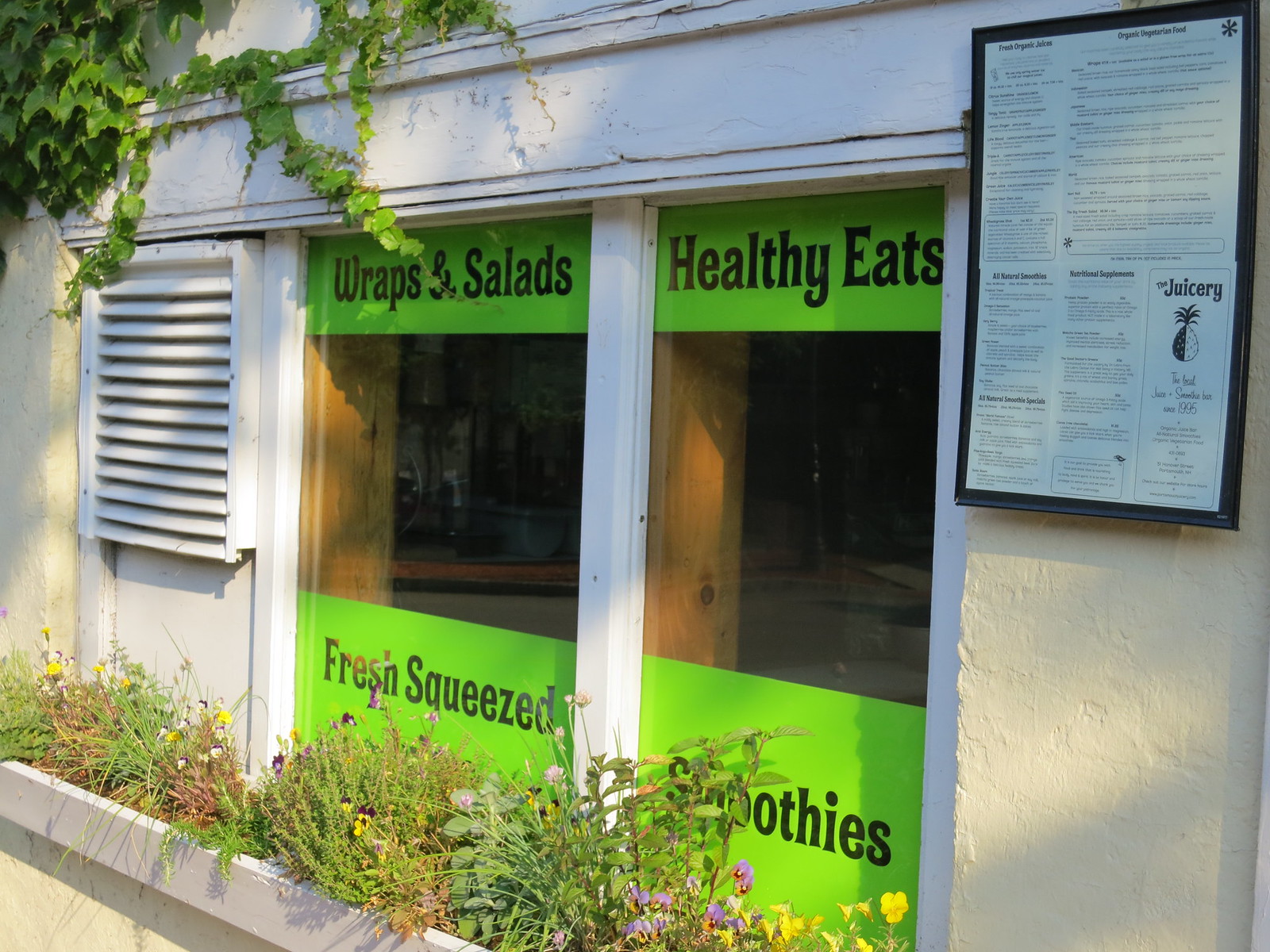The image depicts the front of a small restaurant building with two prominent windows. Each window features vibrant green signs with black lettering. The top left sign reads "Wraps and Salads," while the top right sign says "Healthy Eats." Below each window, the signs display "Fresh Squeezed" on the left and "Smoothies" on the right. A black-framed menu with white text is posted to the right side of the right window, although the text is too small to read. To the left of the windows, there's a vent. Above the windows, the roof is adorned with green plants growing over it like ivy. Below the windows, a flower box bursts with colorful blooms, some of which climb up into the signs. The photo is taken from a slight angle and clearly shot during the daytime, emphasizing the words on the signs and the earthy, vibrant tones of the setting.